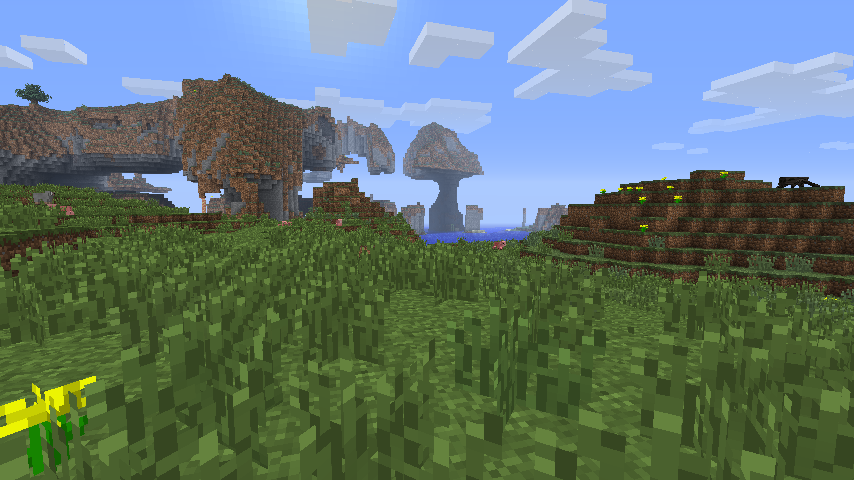The image is a computer-generated scene that looks reminiscent of the game Minecraft, featuring an angular, pixelated landscape. The bottom half showcases a lush terrain made up of green, grassy blocks interspersed with dots of yellow and pink flowers. A terraced area of brown cubes with flat, green tops and patches of yellow flowers appears prominently toward the right. On top of a hill to the right, a small figure, possibly a Minecraft creature, is perched, surveying the landscape. The sky above is a clear blue, dotted with square and rectangular white clouds. In the far background, brilliant turquoise blue water stretches out, with tall, gray and brown rock formations and islands rising from it, including a T-shaped or tree-like mountain formation.